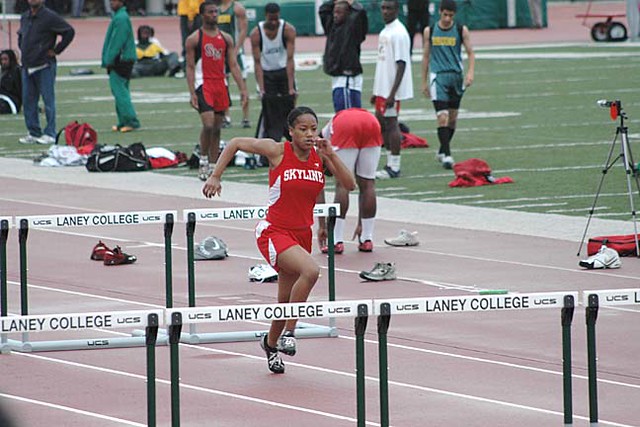In this vibrant, mid-day outdoor photograph taken at a sports track, a woman wearing a red and white tank top with "Skyline" emblazoned on her chest and matching white and red shorts is captured mid-stride, running towards a section of hurdles that read "UCS Laney College." She is positioned centrally in the image, running in the third lane from the left. The track is made of a rubber-like material with painted markings, and various objects, such as scattered shoes, are visible beyond her lane and towards the grass on the right. The background reveals a diverse scene with multiple individuals, some bending over, some walking around, and others standing on what appears to be a football field. A camera is set up to the right side of the track, further indicating the event's organized nature. The colors in the image are rich and varied, hinting at the lively atmosphere of a sports meet. The setting is brightly lit, suggesting that the photo was taken on a clear, sunny day.